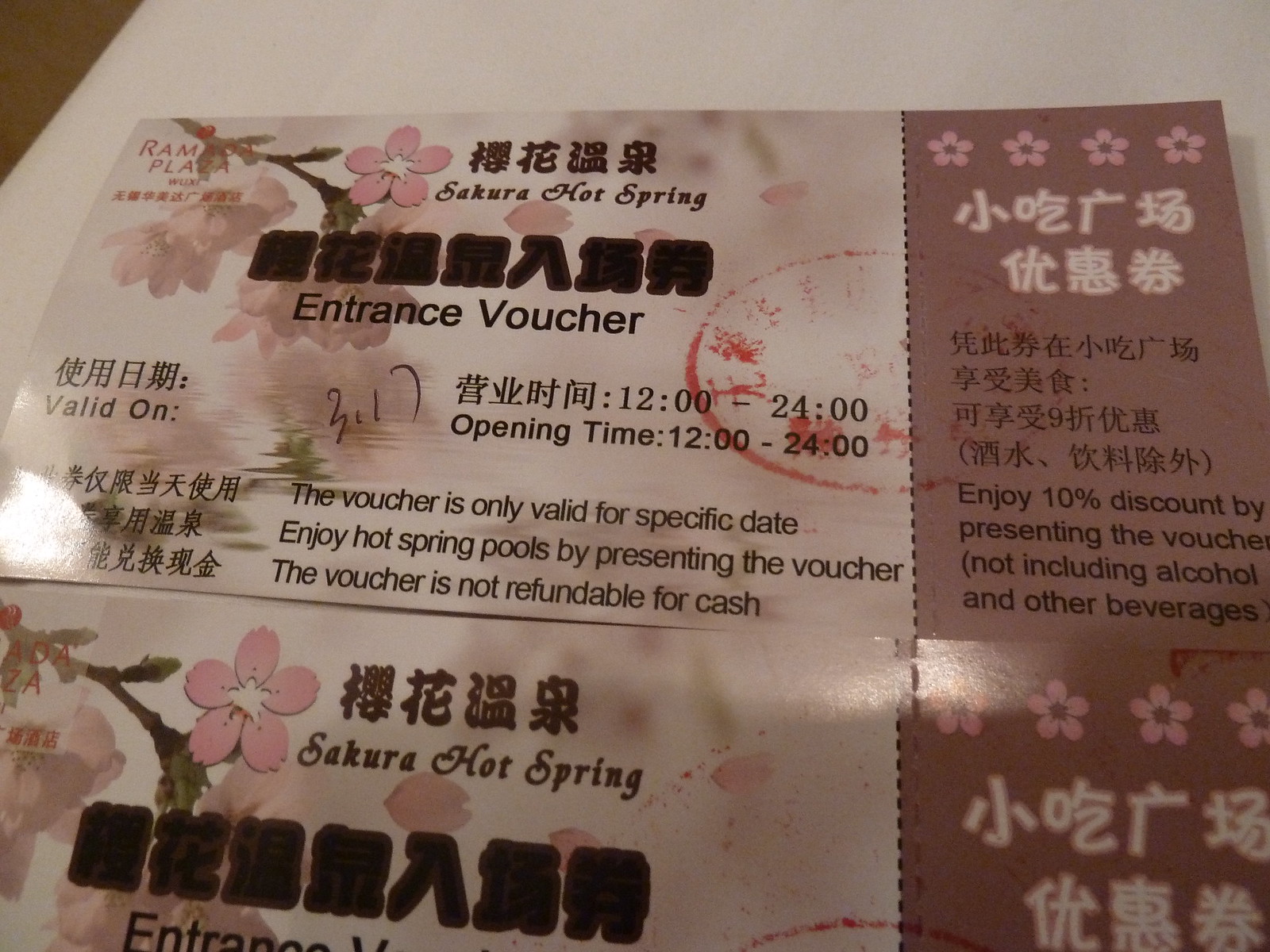The image features two identical laminated entrance vouchers for Sakura Hot Spring, with one slightly overlapping and partially obscuring the other. These vouchers, adorned with a background of cherry blossoms and a clear, watery area, have black text on a pink and white floral backdrop. Each voucher prominently displays the text "Sakura Hot Spring Entrance Voucher" along with the opening times "12:00 to 24:00." There is a red stamp with oriental characters on each voucher, indicating authenticity.

The right side of the voucher includes a vertical perforated line, suggesting a tear-off section. This section states a 10% discount offer, applicable by presenting the voucher, excluding alcohol and other beverages. Additional details specify that the voucher is only valid for a specific date and not redeemable for cash. The upper left corner highlights the Sakura Hot Spring logo, while additional information in both Chinese and English is scattered throughout. The overall aesthetic is very delicate and inviting, reminiscent of a high-end spa or beauty salon advertisement.